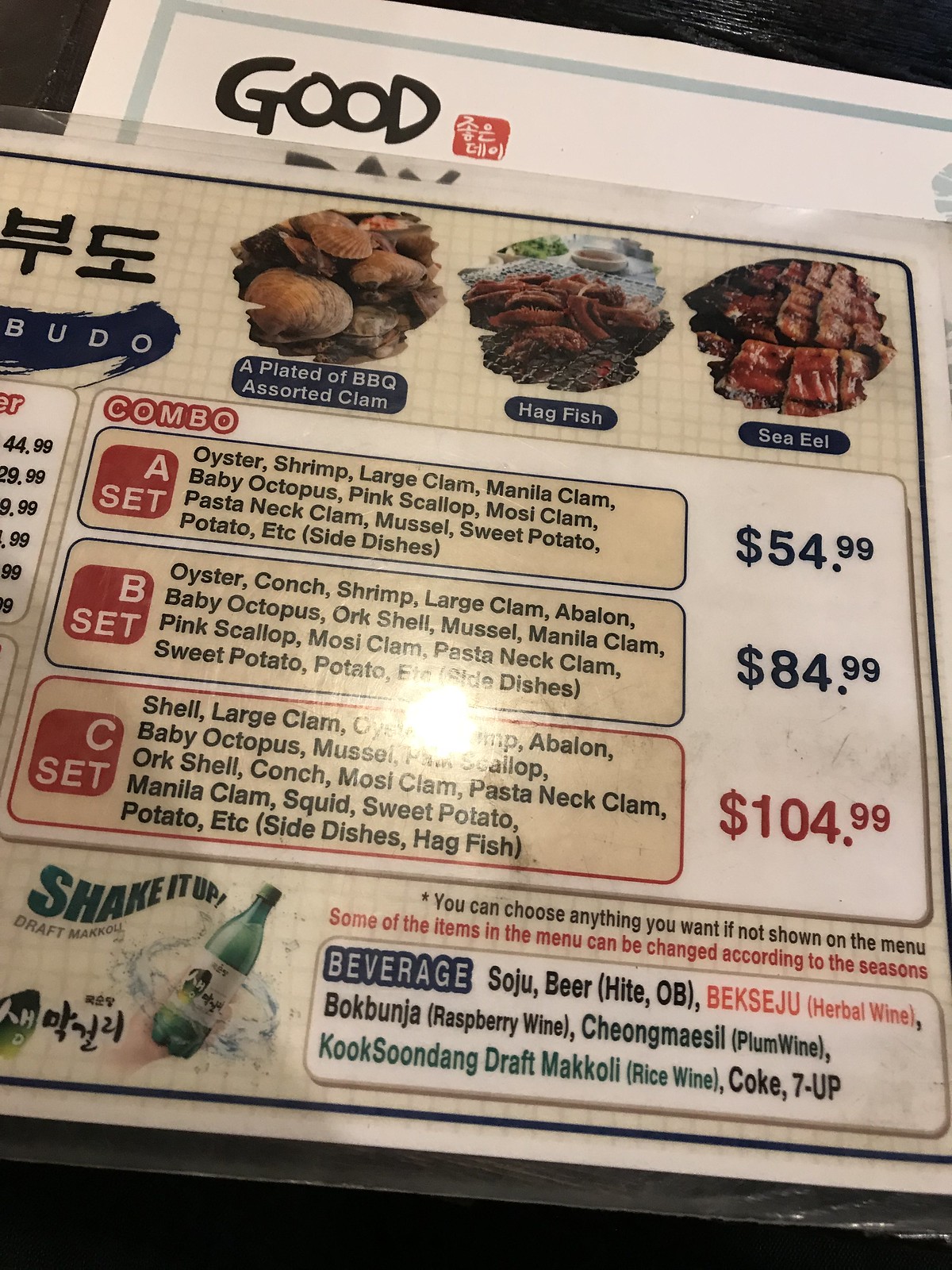This detailed photograph captures part of a restaurant menu and highlights various seafood dishes and combination sets available for dining. At the top of the menu, there are vivid photographs of three meals:

1. A plate of BBQ assorted clam, depicted with multiple clam shells.
2. A serving of hagfish.
3. A dish of sea eel.

The left side of the menu is not visible in this photograph, but the right side, which lists the combos, is in clear view:

- **A Set**: This combo includes oyster, shrimp, large clam, manila clam, baby octopus, pink scallop, mosey clam, pasta nut clam, mussel, sweet potato, potato, and other side dishes, priced at $54.99.
  
- **B Set**: This set features oyster, conch, shrimp, large clam, abalone, baby octopus, orc shell, mussel, manila clam, pink scallop, mosey clam, pasta nut clam, sweet potato, potato, and other side dishes, for $84.99.
  
- **C Set**: This premium combination includes large clam, oyster, shrimp, abalone, baby octopus, mussel, pink scallop, orc shell, conch, mosey clam, pasta nut clam, manila clam, squid, sweet potato, potato, other side dishes, and hagfish, priced at $104.49. Notably, the price for this set is written in red text.

The menu also states that diners can choose items not listed in the menu, and some items may vary according to the season. 

Additionally, the beverage section features a variety of drinks, including soju, herbal wine, raspberry wine, plum wine, rice wine, Coke, and 7-Up.